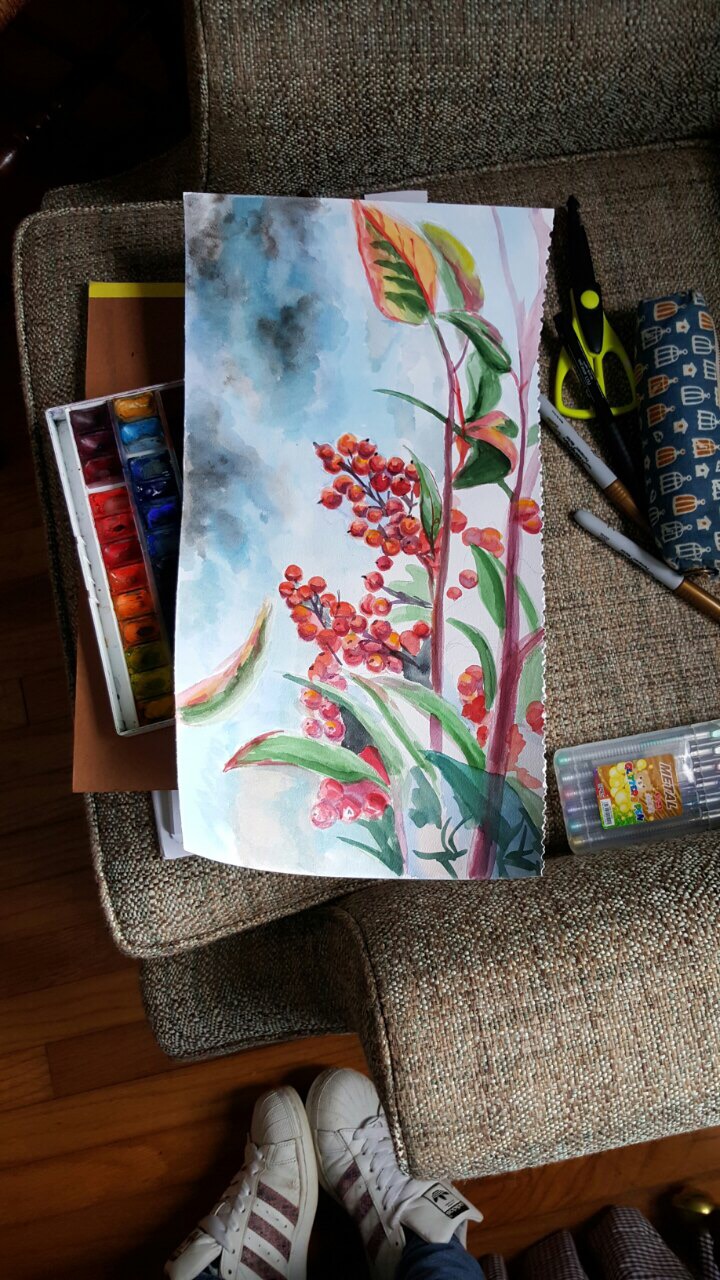A photo taken from above shows a busy workspace with various artistic supplies and personal items. Central to the image is a tall rectangular painting featuring a gradient background transitioning from light blue to dark blue, with a plant bearing red berries and green leaves with pink hues. The painting rests on what appears to be chair cushions which are identified as possibly being part of a tan or gray sofa chair. 

Below the painting, there's a white paint palette smeared with various colors, indicating recent use. Additionally, there are packages: one possibly containing markers and another a box of pencils. The image also captures a pair of black scissors with yellow handles situated to the upper right of the cushions alongside a couple of random pens and small items resembling cigarettes or pipes. Toward the bottom of the image, a pair of white sneakers with black lines or gray stripes and blue jeans are visible, suggesting the presence of the artist. The setup rests on a wooden floor, adding a touch of warmth to the scene.